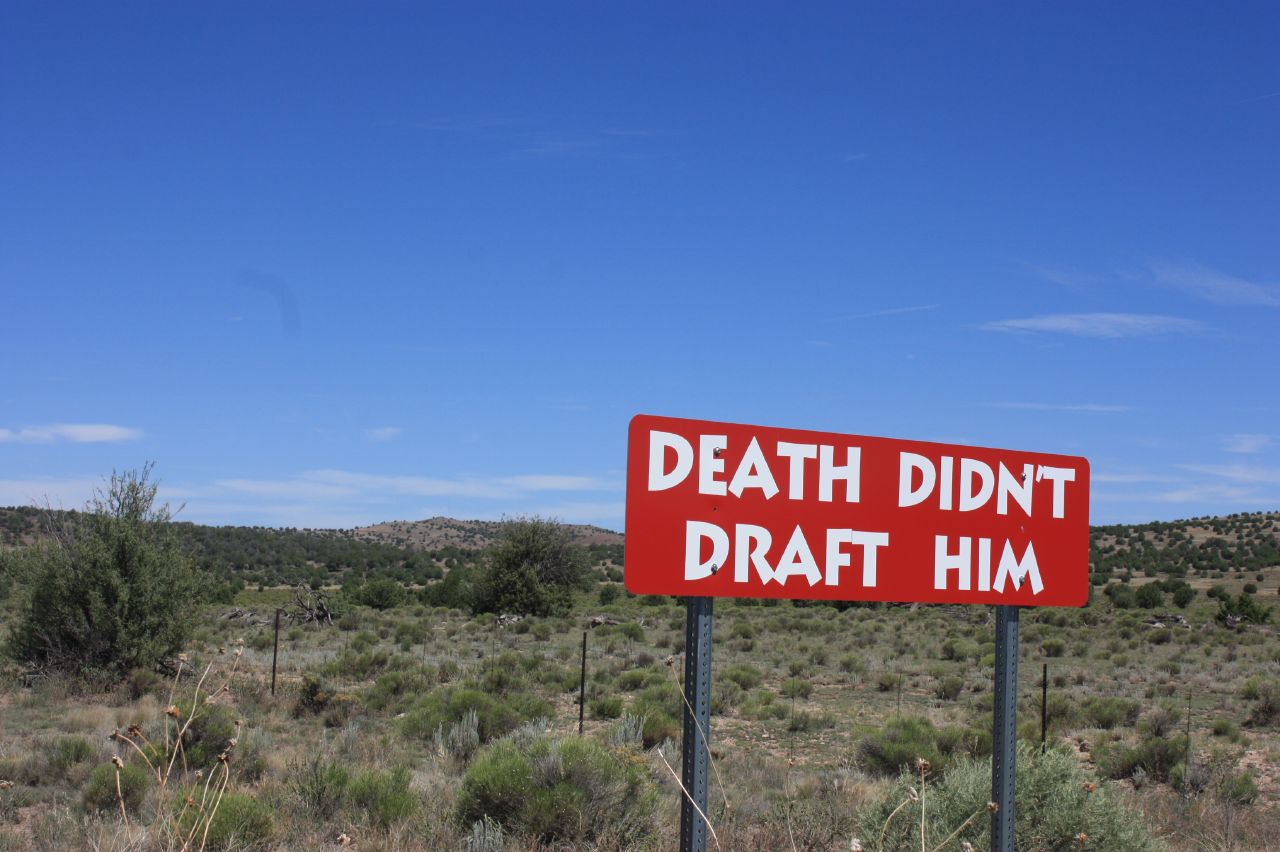In the middle of a vast, barren desert landscape, a striking red sign stands out, mounted on two sturdy gray metal supports. The sign boldly declares in white lettering: "Death didn't draft him." Surrounding this lone marker, the arid expanse is dotted with scattered tumbleweeds and sparse desert vegetation. There are no visible structures or roads nearby, only the undulating desert stretching out as far as the eye can see, with distant hills providing a faint backdrop. A temporary, see-through fence with green supports can be spotted nearby, outlining a patch of this desolate terrain. The juxtaposition of this vivid sign against the endless, monotonous desert creates a haunting and surreal tableau.